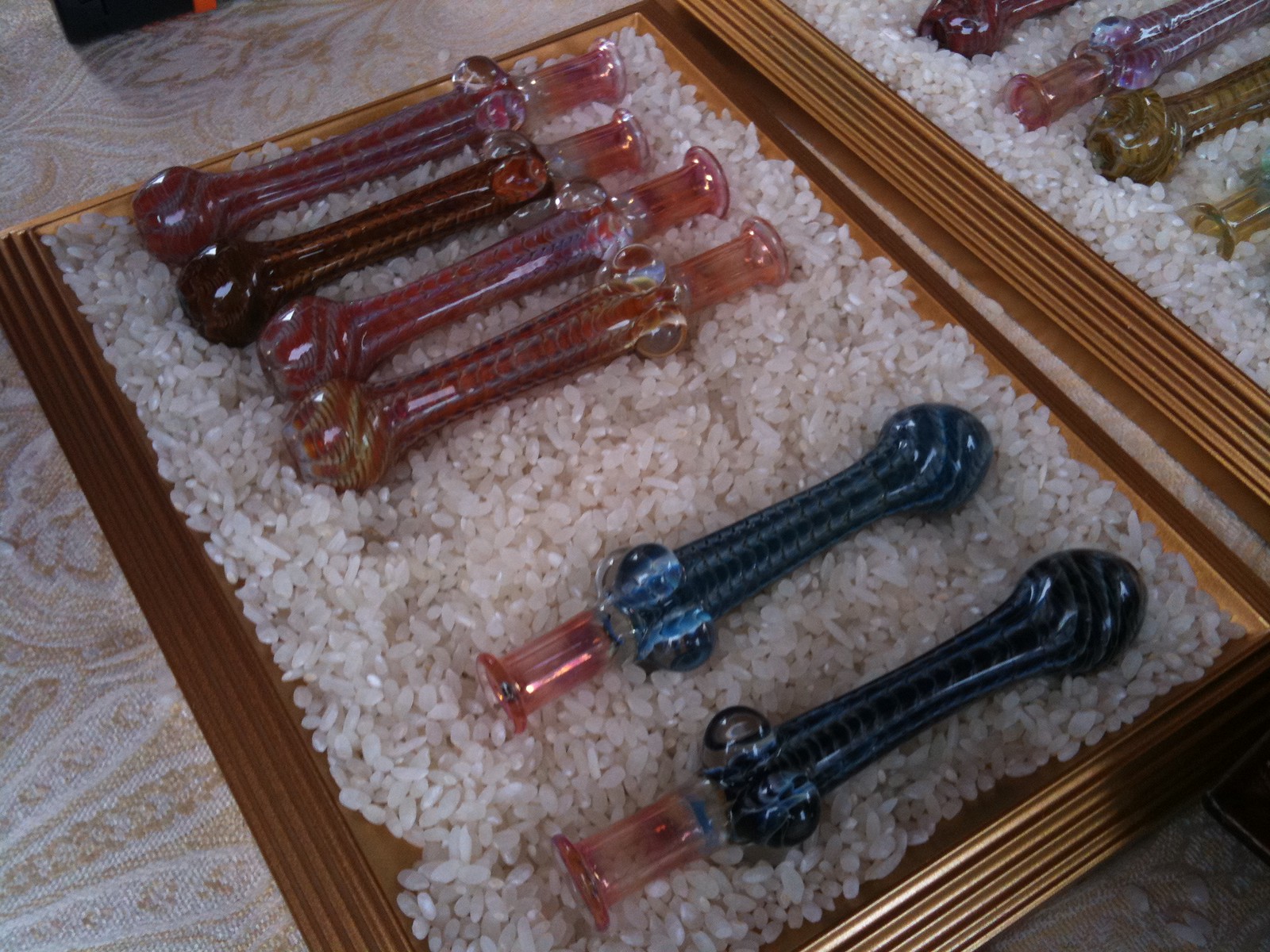Resting on a light beige and white floral-patterned tablecloth is a brown open box filled with white rice. In this box lie six ornate glass objects. Two of them, positioned diagonally in the lower section, have blue bodies with pink tips and rounded bulbous points. The remaining four, situated above the blue ones, are pinkish-red with rounded bottoms and intricate spherical designs around the neck. The overall setup gives the impression of decorative bottle stoppers or possibly vials. At the top right corner, partially visible under another layer of rice, lies another similar box, revealing bits and pieces of three more glass stoppers. The scene is delicately framed in a golden hued border, enhancing the elegant presentation of the glass objects.